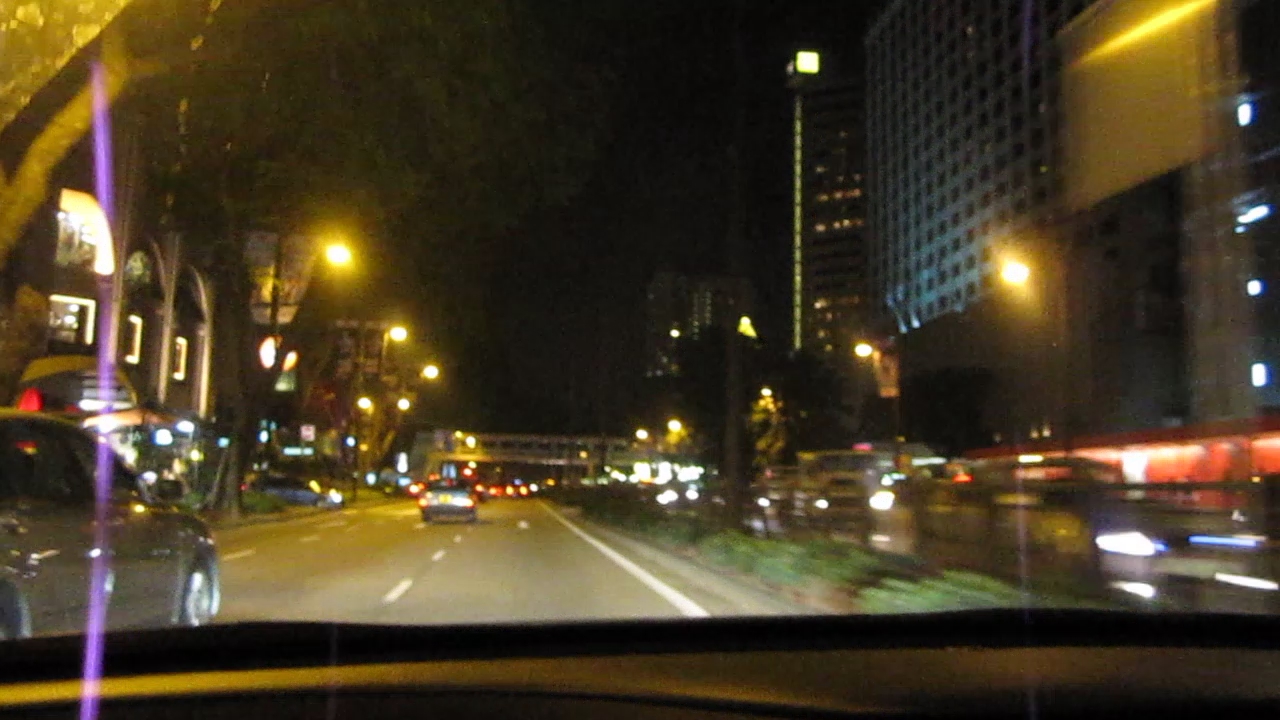This image captures the perspective of a driver traveling down a busy, three-lane road at night. The photograph is taken from inside the vehicle, through the windshield, and the interior of the car is subtly illuminated with a light yellow hue, accented by a purple streak from light reflections. In the rightmost lane, where the driver's car is located, the traffic is ongoing, moving at a noticeable speed, causing some motion blur. To the driver's left, the middle lane accommodates two visible vehicles: a gray car directly adjacent and another further ahead, marked only by its taillights. A grassy strip with streetlights and poles divides the road, and the leftmost lane has incoming traffic.

On both sides of the road, numerous towering buildings are lit up, their predominant white lights occasionally interrupted by yellow hues and some red lights near their bases. These buildings comprise both business establishments and apartment complexes. Farther ahead, an elevated pedestrian bridge spans across the road, ensuring safe passage for those on foot. The presence of streetlights lining the road aids visibility, and the entire scene is framed by the bustling urban skyline surrounding this lively avenue.